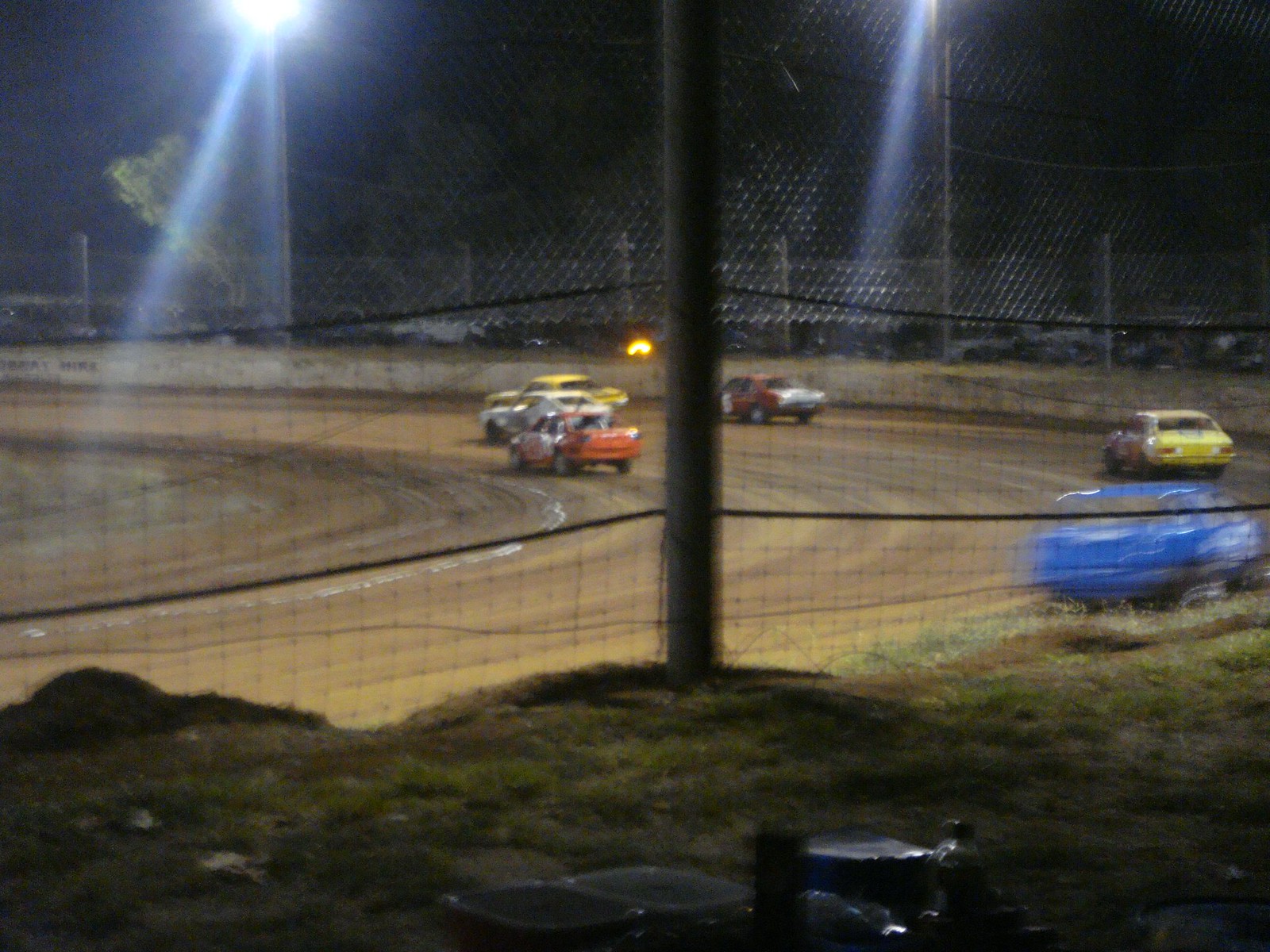The image captures a nighttime scene of a dirt racetrack, featuring a localized race event. In the photograph, six cars can be seen making a left-hand turn on the track, which is a mixture of green and brown surfaces. The shot is taken from behind the racing field, highlighting a large fence that encircles the track. The upper half of the fence is made of chain-link, while the lower part consists of wires arranged in a square pattern, all attached to poles. There is a patch of grass at the bottom of the image, slightly elevated above the racetrack. Bright lights illuminate the field from both the left and upper right, adding to the dramatic nighttime setting. Trees are visible in the background, contributing to the natural, outdoor feel of the racing event.